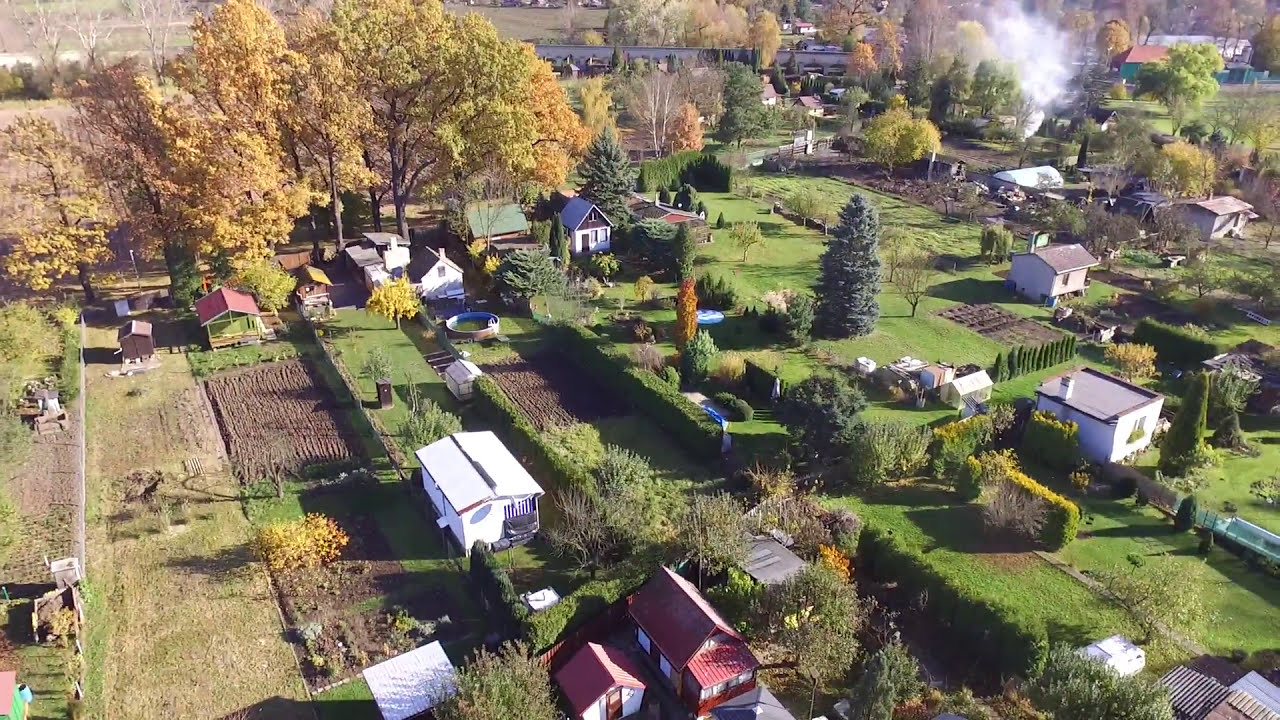An aerial, overhead shot captures a picturesque, rural Midwestern town, possibly taken using a drone. The landscape reveals a meticulously organized small community, characterized by various small farmhouses peppered through lush greenery. The houses, which come in different shapes, sizes, and colors, are dotting the area amidst a tapestry of long, narrow garden plots and parcels of tilled soil. Many homes feature well-maintained backyard gardens, some enclosed by square hedgerows, showcasing neat rows of tilled soil. Autumn has touched the landscape, as seen by the yellowing leaves on the trees, particularly in the top left corner where large orange trees stand out.

Further enhancing the scenery’s rustic charm, the background features expanses of green grasslands and more clusters of trees. White smoke rises in the top right corner, partially obscured by trees; it’s unclear if it’s emanating from a chimney or a possible controlled burn, adding a hint of activity.

In the town center, a small red house stands near a small white one, surrounded by fences and hedgerows, with other white buildings behind them. The community has a well-ordered grid layout, with bright green grasses, scattered sheds, and some uniquely shaped features, like a round swimming pool centrally located. This aerial view captures not only the intricate organization of the gardens and homes but also the tranquil and quintessentially rural essence of this Midwestern town.